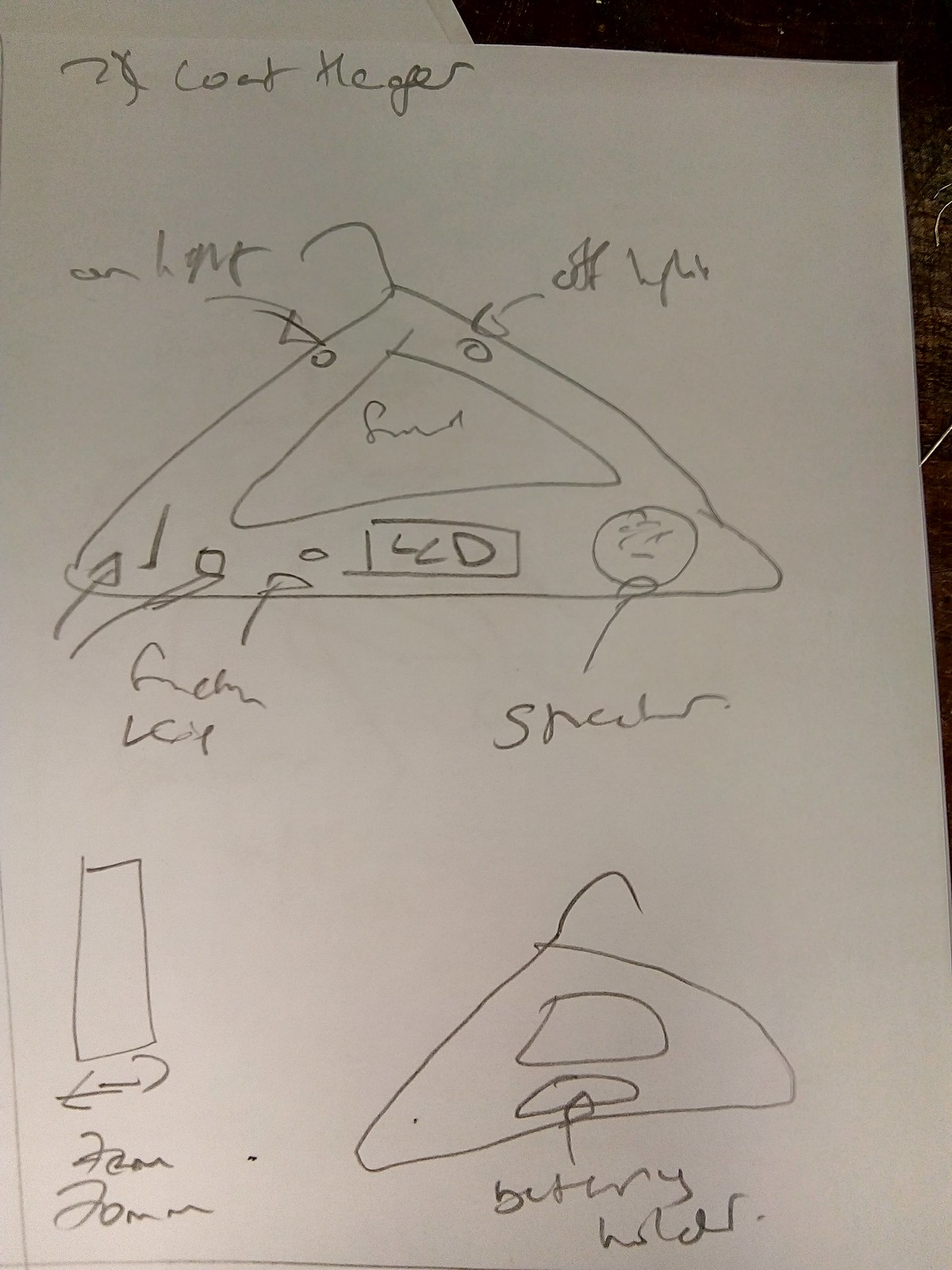This image features a detailed pencil drawing on a piece of white paper, oriented in portrait format. 

### Top Half:
- **Main Drawing**: The primary focus is a meticulously rendered pencil sketch of a coat hanger. The hanger exhibits a classic triangular shape with a half-oval hook emerging from the top.
- **Labels and Arrows**: Various features of the hanger are annotated with words and arrows pointing to specific sections. Although the labels are difficult to decipher, one can observe that both the top part of the triangular structure and the base of the hanger include detailed annotations, particularly highlighting two holes situated near the top.

### Bottom Half:
- **Secondary Drawing**: Below the main sketch is a smaller depiction of a coat hanger. This drawing is accompanied by the description "Better Holder," indicating an improved or alternative design.
- **Rectangular Label**: Adjacent to this smaller hanger illustration, there is a small rectangle labeled "20 millimeters," potentially specifying a dimension related to the hanger design.

### Additional Notes:
- **Text at the Top**: At the very top of the paper, the phrase "Two Times Coat Hanger" is written in pencil, possibly denoting that the drawing represents two iterations or versions of the coat hanger.
- **Background and Tools**: The paper is placed on what seems to be a dark wooden table. The entire drawing is executed using a medium gray pencil, without any other colors involved in the artwork.

The composition, annotations, and layout suggest a detailed study or design plan for a coat hanger, with meticulous attention to dimensions and functional aspects.